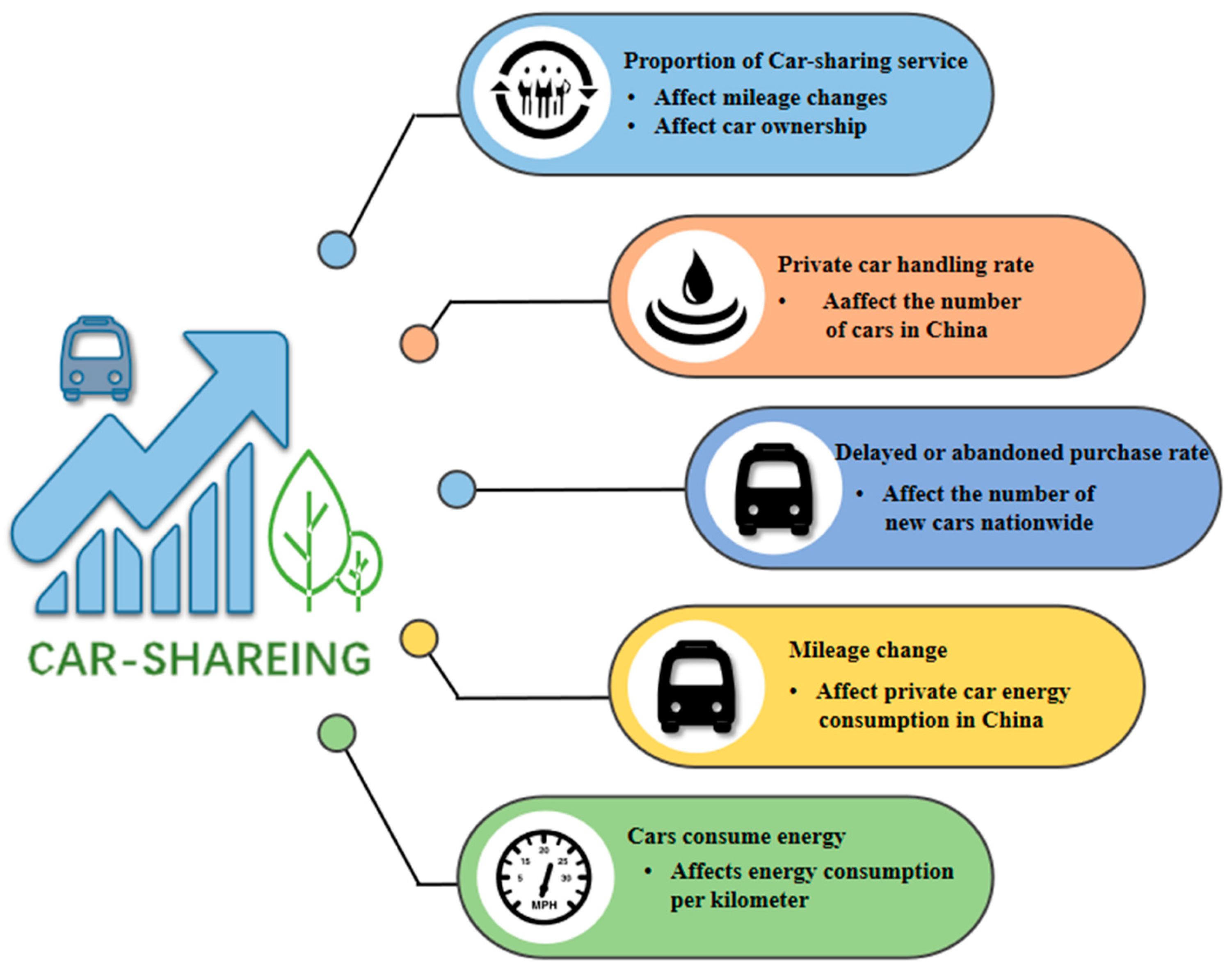The infographic illustrates the impacts of car sharing on various factors related to transportation and energy consumption. On the left side, a jagged upward-pointing arrow graph commonly associated with stock markets or cryptocurrency trends features colorful, rudimentary icons of a car or bus and green trees. Beneath this, the term "car sharing" is prominently displayed. 

To the right, five colored, rounded text boxes with small arrows direct attention toward the car-sharing logo. The light blue box at the top includes an icon of people within a circular arrow, detailing that "proportion of car sharing services affects mileage changes and car ownership." Below, the pink box with a water drop icon discusses how "private car handling rates affect the number of cars in China." The darker blue box, featuring a bus icon, mentions the "delayed or abandoned purchase rate affecting the number of cars nationwide." The yellow box, also with a bus icon, outlines how "mileage change affects private car energy consumption in China." Lastly, the green box at the bottom, showcasing a speedometer icon, notes that "cars consume energy, affecting energy consumption per kilometer."

This ecological-style infographic, likely designed for a PowerPoint presentation, emphasizes how increased car sharing influences people's behavior, the quantity of cars on the road, and the broader implications on the transportation and energy sectors, particularly in regions like China.